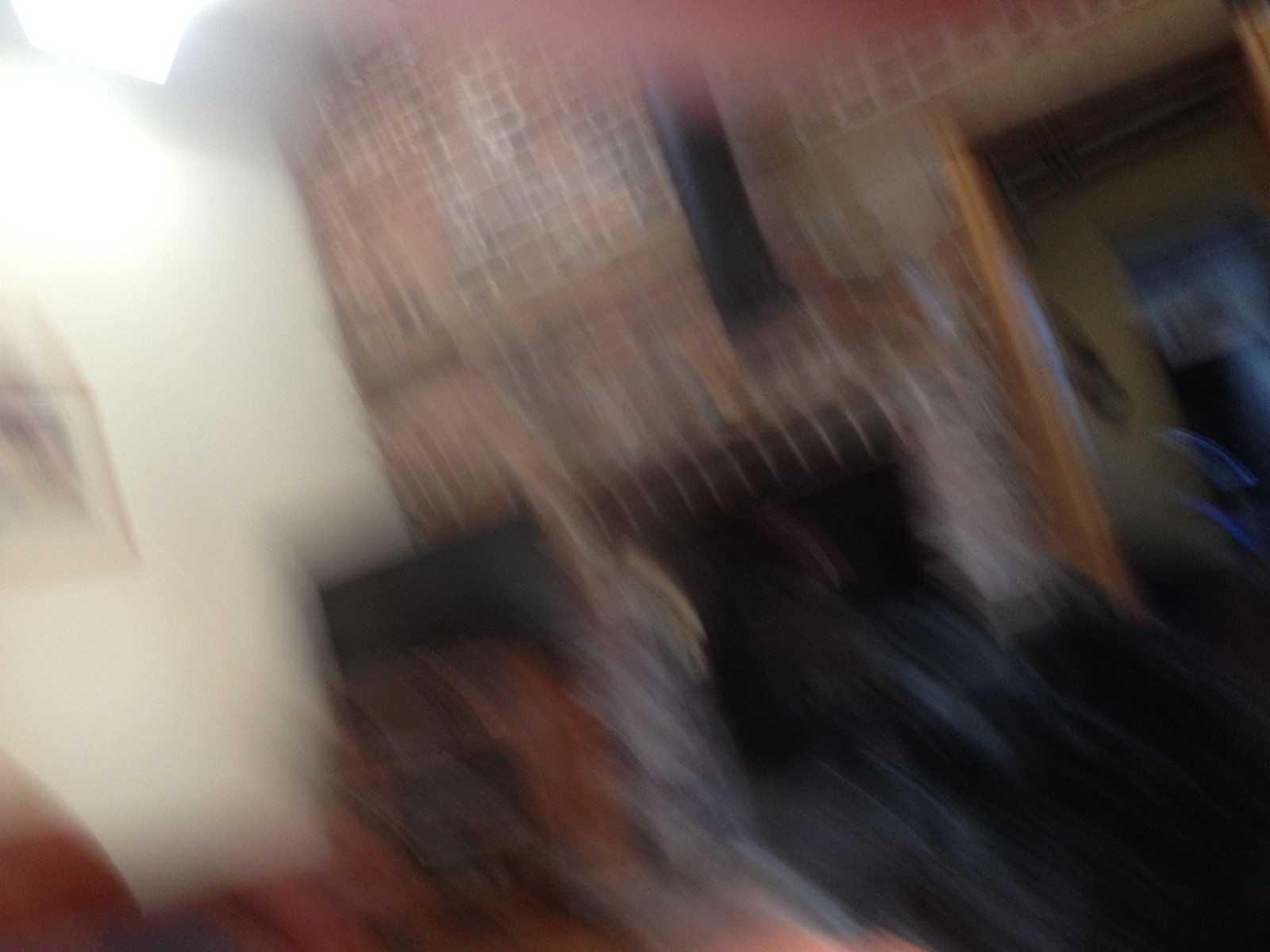The photograph is a completely distorted and out-of-focus image, making it difficult to discern clear details. On the left side of the image, there is a white wall that occupies about a fifth of the frame, with a faint silhouette suggesting a picture or photograph hanging on it. Adjacent to the white wall, at a right angle, there's a red brick wall featuring a possible doorway or mirror outlined in black. This brick wall is identified in the top right corner of the photograph. Below, there are indistinct black and red shapes that might be shadows or possibly people sitting, adding to the overall impression of the image's foreground. The bottom of the photo shows streaks of gray, black, white, and rust-colored orange. Additionally, there is a patch of bright light reflecting off an object in the upper left corner. The main focal points seem to be the distorted brick wall, the opening on the right side leading to another room, and the shadowy figures possibly occupying the center of the image.